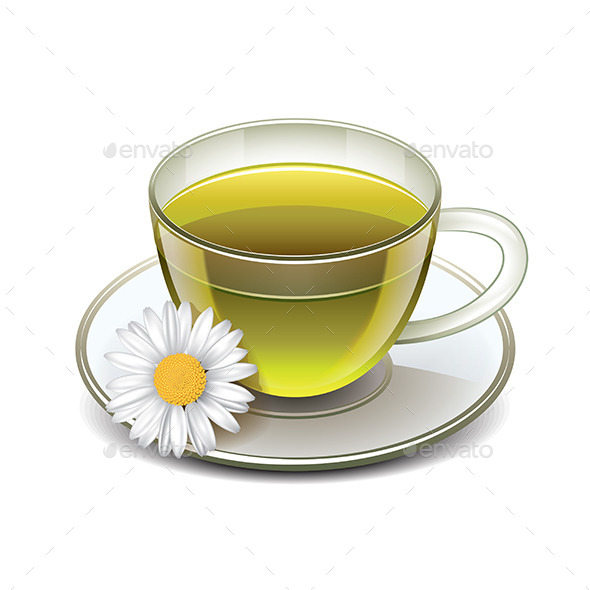In the center of this image is a detailed, computer-drawn depiction of a clear glass teacup with a curved handle, filled with a translucent light green liquid, likely green tea. The cup sits atop a clear, round saucer, and near the edge of the saucer rests a daisy with white petals and an orange-yellow center. The entire illustration is set against a white background with faint crisscrossing lines. Subtly embedded in the background pattern is a gray watermark that reads "Envato," accompanied by a small emblem resembling a closed hand, discreetly positioned just before the 'E' in the text. The overall colors in the image include various shades of white, along with hints of yellow, lime green, brown, and some black edging around the teacup. This stock image appears perfectly centered, likely intended for use in digital and web-based designs.